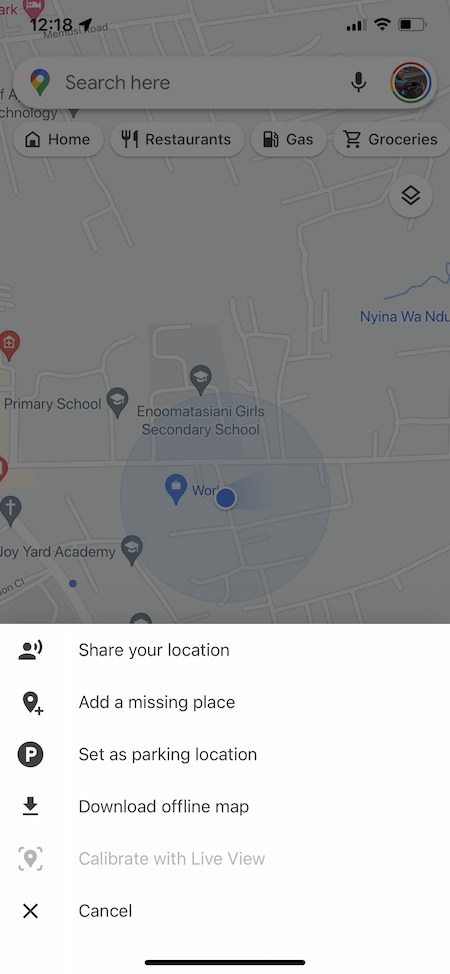A detailed screenshot from a smartphone displays a Google Maps interface. In the upper left-hand corner, the time reads 2:18. The device status icons show three bars of cellular signal strength, an active Wi-Fi connection, and a battery at half charge. The Google Maps search bar is currently empty. Below the search bar, quick access options are available for Home, Restaurants, Gas, and Groceries. The map view highlights several locations, including a primary school, an academy, and Inumatase'ani Girls Secondary School. At the bottom of the map interface, there are additional options, such as sharing your location, adding a missing place, setting a parking location, downloading an offline map, calibrating with live view, or canceling actions. A prominent black horizontal line marks the bottom edge of the screenshot.